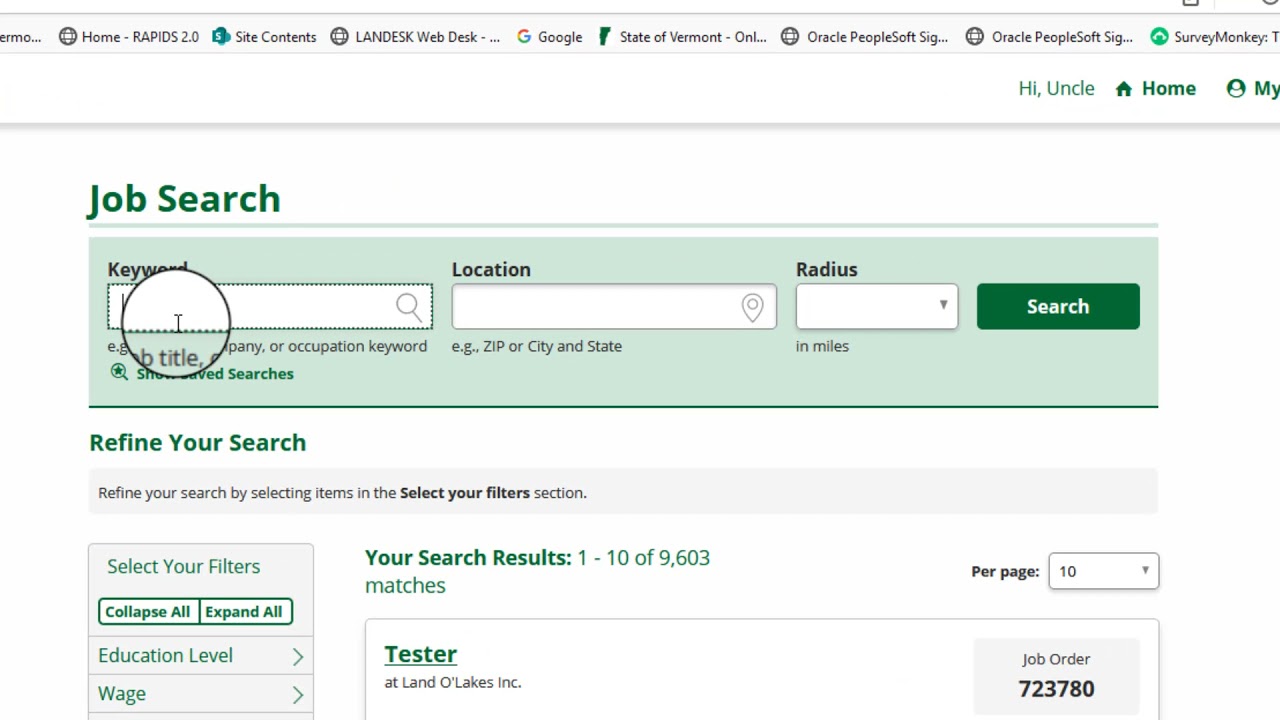The image captures a partial view of a web browser displaying a website. The browser window, which is roughly 30% to 50% wider than it is tall, features a bookmarks bar at the top occupying approximately 5% to 10% of the screen's height. The bookmarks bar includes shortcuts to various sites like Home, Rapidus 2.0, Site Contents, LANDESK, Web Desk, Google, State of Vermont, Oracle PeopleSoft (listed twice), and SurveyMonkey.

Beneath the bookmarks bar, there is a white section transitioning into a gray bar that together take up about 15% of the screen's height. To the right within this section, although partially obscured, there is dark green text that reads "Hi, Uncle" next to a small house icon labeled "Home" and a person icon partially showing "My."

The main content of the site is centered below this gray bar. On the left, slightly indented, is a large, dark green heading that reads "Job Search." Under this heading, several search fields are visible alongside a search bar located to the right. At the very bottom of the section, the search results are displayed. The right side of the screen appears to be cut off, hiding some details from view.